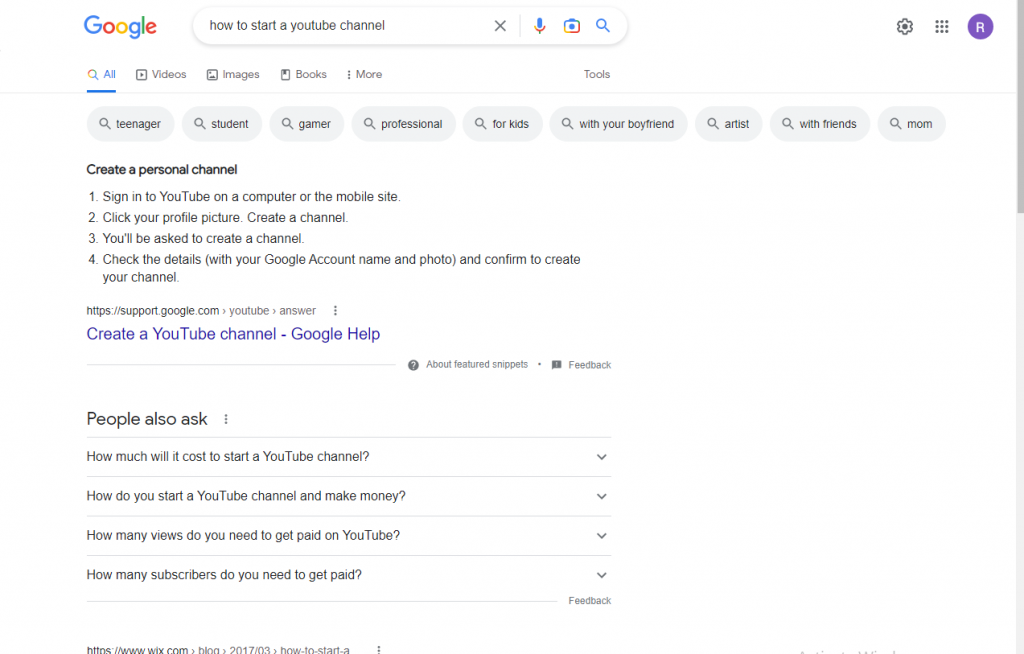The image displays a Google search results page for "how to start a YouTube channel." On the left, the familiar Google logo is prominently featured, while on the right, there is an 'X' button to close the search. Moving to the extreme right, icons for a microphone, a camera lens, a magnifying glass, and a gearbox with a grid of dots line up sequentially. The user is logged into an account identified by a purple circle containing the initial "R."

Just below the Google search bar, there are menu options including "All," "Videos," "Images," "Books," and "More," with "All" highlighted in blue and underlined. To the right, beneath the magnifying glass icon, there’s a "Tools" option, also highlighted in blue.

Further down, the search results begin. The first section presents various specific search suggestions like "teenager," "student," "game," "professional," and "for kids." Below these suggestions, a detailed guide outlines the four steps to creating a personal YouTube channel:
1. Sign into YouTube on a computer or mobile site.
2. Check your profile picture and select "Create a channel."
3. Follow the prompts to create your channel.
4. Review the details with your Google account.

A link to additional resources and Google's help page for creating a YouTube channel is provided at the bottom of this guide. To the right of this guide snippet, there is a question mark icon that offers more information about featured snippets along with a feedback option.

Also displayed are questions commonly asked by users under the "People also ask" section, such as "How much does it cost to start a YouTube channel?", "How do you start a YouTube channel and make money?", "How many views do you need to get paid on YouTube?", and "How many subscribers are required to get paid?" Each of these questions can be expanded to reveal more information.

The entire interface is set against a white background, maintaining the clean, minimalistic look typical of Google's design.